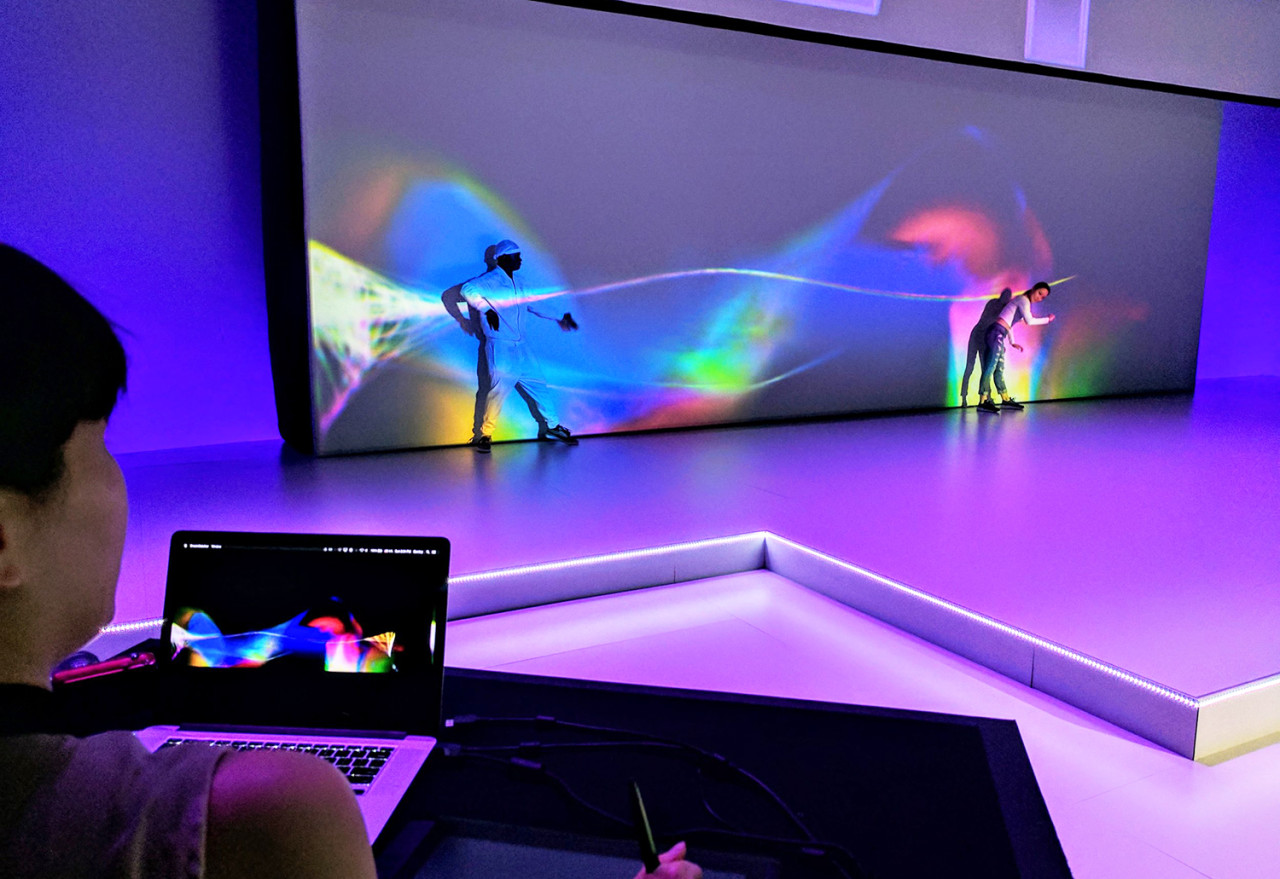In a captivating scene, a person operates a MacBook, which displays vibrant neon colors in blue, pink, and green, arranged in a linear pattern. This imagery is projected onto a large, modern white stage with a sizable movie-style screen that mirrors the neon hues from the laptop. On the stage, two performers dressed in white, one man standing and another bending over slightly, are illuminated by the neon rainbow that stretches across their bodies. The man wears urban attire including a do-rag and sweats, enhancing the contemporary vibe of what appears to be a dynamic dance performance. The expansive screen behind them not only projects the neon light but also their shadows and reflections, adding an artistic dimension to the scene. The encompassing lights shift from light yellow to blue to green, creating a mesmerizing ombre effect that adds to the ambiance of what seems to be an elaborate art show.